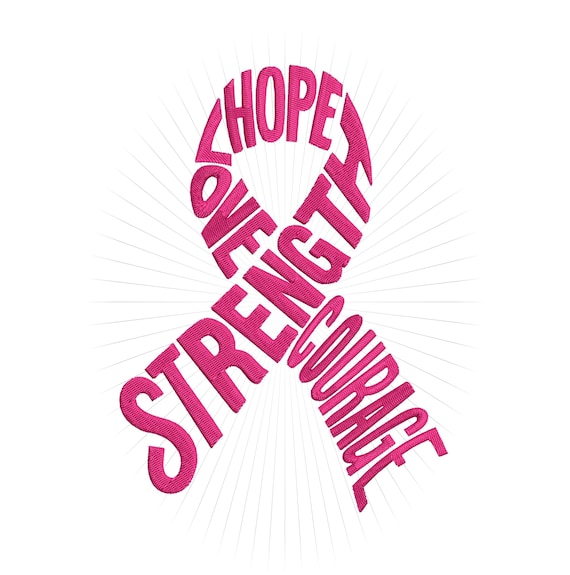The image is a detailed clip art-style drawing of a breast cancer awareness ribbon. This pink ribbon, typically a symbol of support for breast cancer patients and survivors, is uniquely formed from the words "strength, hope, love, courage." The letters, rendered in a vibrant magenta, create the recognizable loop shape of the ribbon. Each letter is cross-hatched with black for added texture and variation in size and shape, giving the ribbon a dynamic, three-dimensional feel. Surrounding the ribbon, pale gray lines radiate outward, symbolizing the spreading of these positive attributes. The entire composition is set against a plain white background, accentuating the simplicity and poignancy of the message, making it a striking and uplifting icon likely intended for use in ads, medical settings, or support materials.